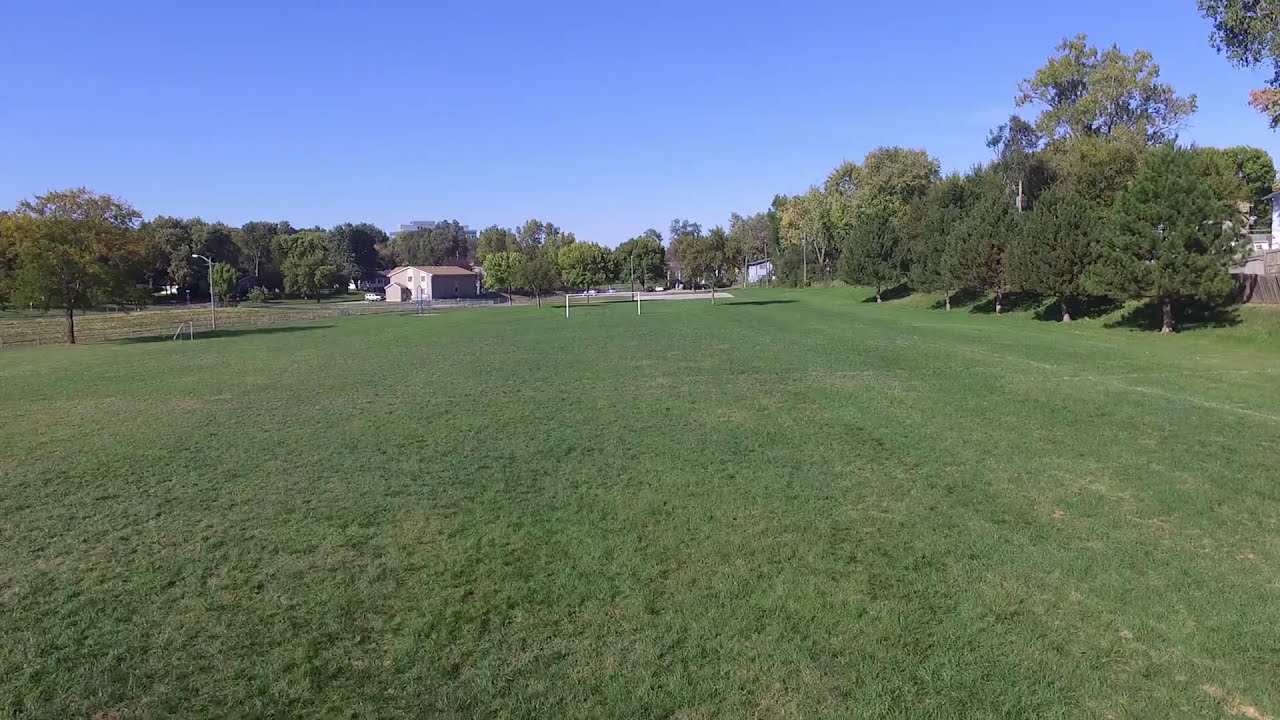The photograph captures a beautifully maintained green field that appears freshly mowed, with only occasional glimpses of brown ground between the blades of grass. The field stretches out flat from the foreground to the horizon. Lining the left and right sides are lush trees, providing a natural boundary. On the right edge, a row of neatly planted pine trees adds a touch of organization to the otherwise wild scenery.

At the back left of the field, around 50 feet from the camera, stands a modest beige house, enhancing the landscape's residential charm. The house seems to be approximately 200 to 300 meters away from the farthest point of the camera’s elevated view, which is angled to keep the ground parallel to the lens.

Beyond the house, rows of tall trees form a natural horizon line, emphasizing the depth and openness of the area. The field contains metal goalposts, hinting at recreational use. The sky is a brilliant, clear blue, unmarked by clouds, creating a serene, inviting atmosphere for the scene.